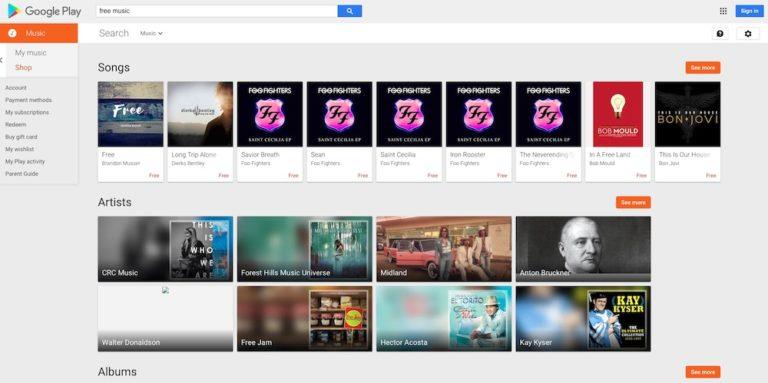The image depicts the Google Play Music interface, showcasing the "My Music" section and the "Music Shop." Below these sections, there is a search bar on the right labeled "Free Music" and a search button. Additionally, the display highlights a song featuring an image of a man silhouetted against a sunset. 

There are also five songs featuring a distinctive pink shield emblem with "FF" on it, representing the band Foo Fighters. Other displayed content includes a red book icon with a light bulb illustration, and a song labeled "Bon Jovi." 

Further listings include music albums from various artists and genres: CRC Music, Walter Donaldson, Forest Hills Music Universe, Free Jam, Midland, Hector Acosta, Anton Bruckner, and K. Kaiser.